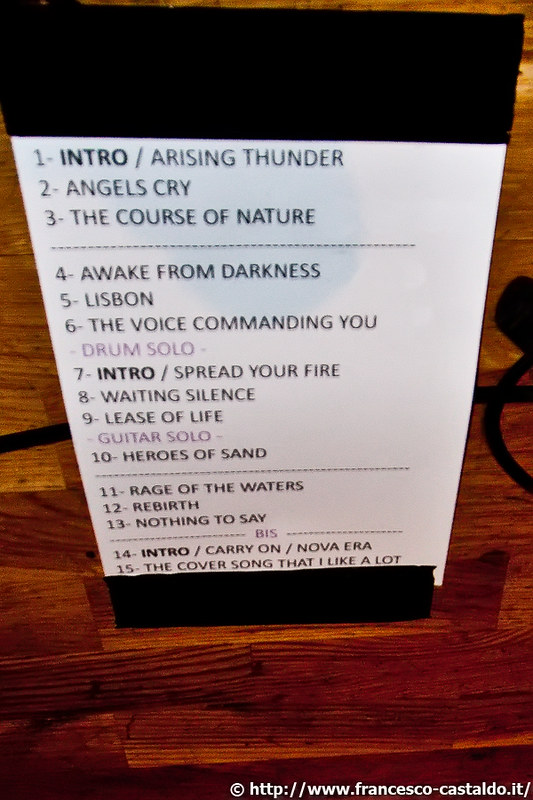The image depicts a meticulously detailed setlist, possibly for a concert or an album, printed on a vertical white sheet of paper. This sheet is secured by broad black tape at both its top and bottom edges and appears superimposed on a dark wooden background, potentially a wall or table. The setlist is numbered from 1 to 15, with entries written in predominantly black text and occasional purple text denoting solos.

1. **Intro / Arising Thunder**
2. **Angels Cry**
3. **The Course of Nature**
4. **Awake from Darkness**
5. **Lisbon**
6. **The Voice Commanding You** (followed by a drum solo in purple text)
7. **Intro / Spread Your Fire**
8. **Waiting Silence**
9. **Lease of Life** (followed by a guitar solo in purple text)
10. **Heroes of Sand**
11. **Rage of the Waters**
12. **Rebirth**
13. **Nothing to Say** (marked with "B.I.S." in purple, flanked by horizontal lines)
14. **Intro / Carry On / Nova Era**
15. **The Cover Song that I like a lot**

At the bottom-right corner of the image, a small white text displays a copyright symbol and the website "www.francisco-castellano.it." The visually clean design, combined with strong black and purple highlights, suggests a thoughtful compilation, possibly personal or professional, documenting a sequence of musical pieces or performance acts.